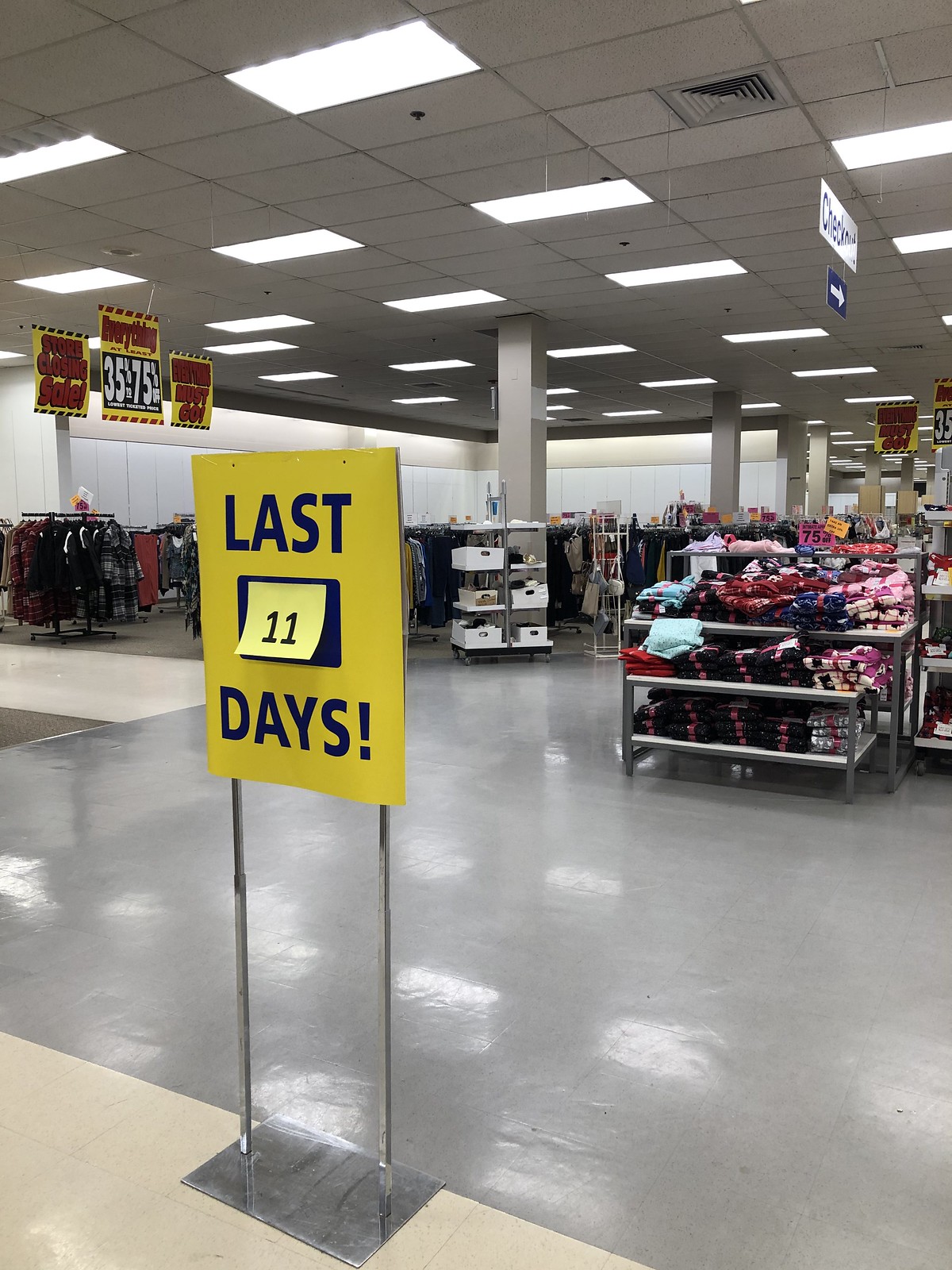The image depicts the interior of a large, possibly big-box, department store that is in the midst of a store closing sale. Dominating the center of the scene is a prominent, vertically rectangular yellow sign, held up by two silver rods anchored to a silver platform. This sign has the words "Last Days" in black lettering, with a black square in the center containing a bright yellow sticky note marked with the number "11." This indicates the final 11 days of the sale.

In the background and foreground, a variety of merchandise is visible, with clothing displayed on both shelves and hangers. Some of the shelves, particularly on the right side, are cluttered with piles of garments. The discount signs hanging from the ceiling inform shoppers of significant markdowns, ranging from 35% to 75% off. The store's ceiling features gray tiles interspersed with recessed rectangular fluorescent lights. The floor is a mix of glossy light gray tiles with some areas of beige tiling. Further back, white boxes are neatly arranged on the shelves. The left side of the frame shows some brown shelving units, adding to the mix of colors in the interior. The overall ambiance reflects a store in its final days, filled with the hustle of a clearance sale.